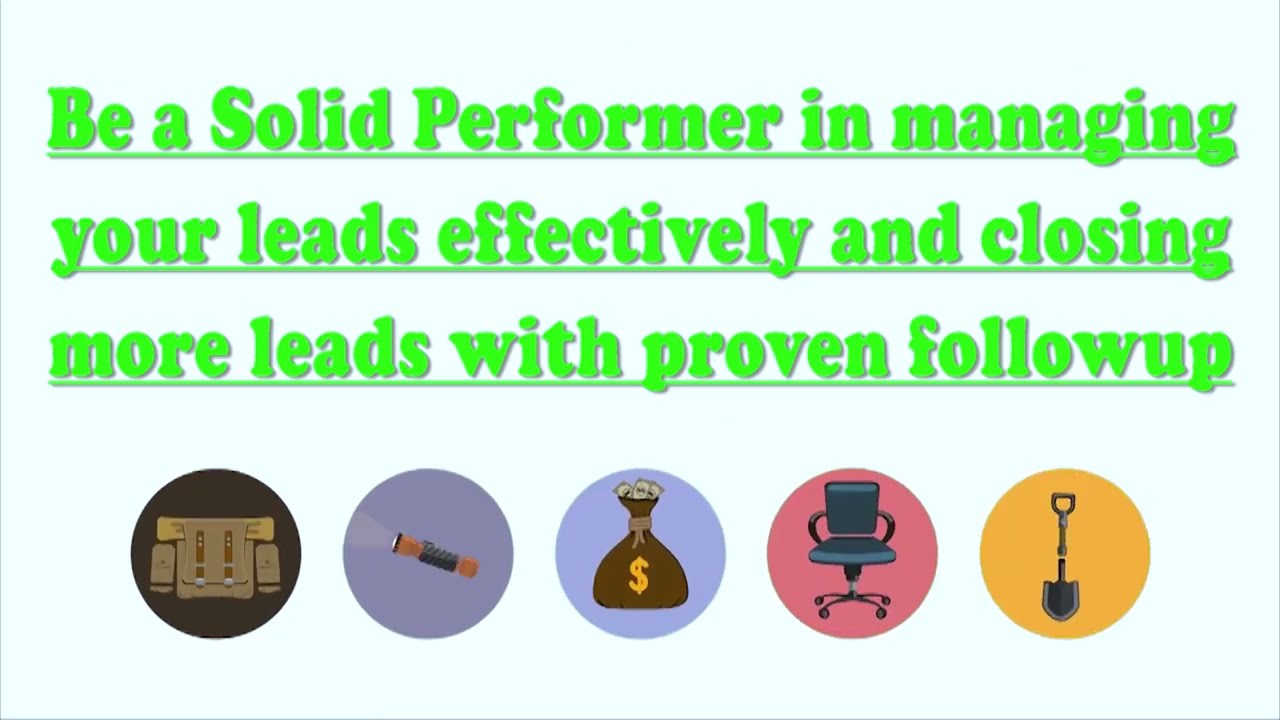This image features a white background framed by a black line on the sides and bottom. At the top, three lines of center-justified, green text with a gray drop shadow and underlined read: "Be a solid performer in managing your leads effectively and closing more leads with proven follow-up." Notably, "Be a solid performer" is capitalized, while the rest is in lowercase. Below this text, there are five circular icons, each with distinct images and colors, arrayed from left to right: a brown circle with a book bag or t-shirt; an orange and black flashlight against a dark purple circle; a yellow money symbol on a brown money bag within a purple circle; a black office chair on a pink circle; and a black shovel in an orange circle.